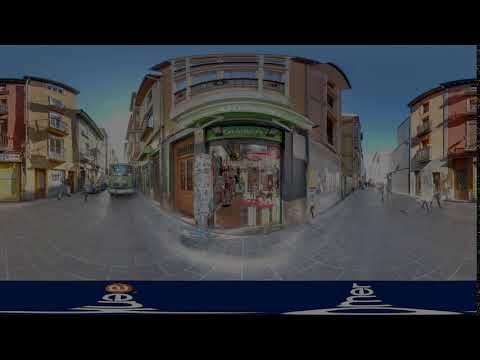This image, seemingly captured through a fisheye lens or a panoramic view, presents a vibrantly colorful town square, possibly from a city overseas like Italy or Denmark. Dominating the scene is a prominent marketplace building, featuring a unique blend of architecture with a brown and green facade, adorned with a green awning and plastered flyers on the doorway. The ground is a mix of concrete pavement and cobblestone streets, bustling with people walking around. To the left, there are interconnected buildings, three to four stories high, showcasing hues of blue-green, yellow, and pink, with numerous windows, indicative of apartment buildings or stores. An SUV or bus, likely green, navigates through the streets amidst parked cars. The sky above is a mostly blue hue, albeit with a muted effect as if filtered, enhancing the scene's animated, almost 3D appearance. Notably, a corner store with a peach and reddish facade is visible, and the entire composition is framed by a blue outline at the bottom, adding a striking contrast to the town's lively atmosphere.